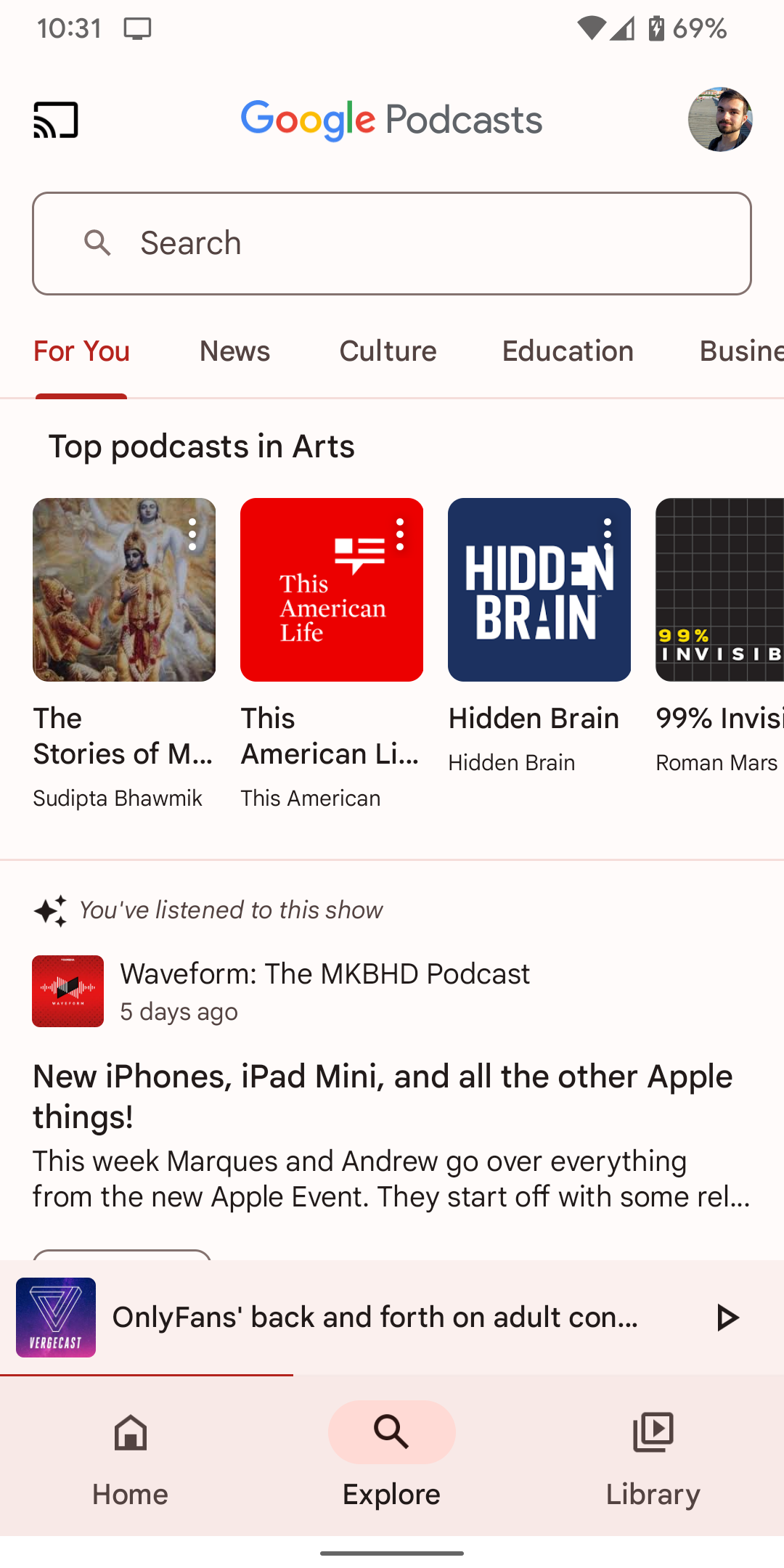This screenshot captures the home screen of a smartphone featuring a light pink background. In the status bar, the current time is displayed as 10:31 AM on the top left corner. On the top right, indicators show the Wi-Fi signal at half strength and the battery at 69%. Below the status bar, there is an icon to enlarge the view. The central area displays the "Google Podcasts" app, with a circular profile picture situated to the right.

Directly beneath, there's a search box featuring a magnifying glass icon with the word "Search" inside. Below the search box, three tabs are visible: "For you," which is highlighted in red, followed by "News," "Culture," "Education," and "Business." A subtle light gray line demarcates the sections underneath.

Beneath this line, the heading "Top Podcast and Arts" introduces four squared thumbnails. The leftmost square showcases a mythical image depicting warriors. To its right, a red square displays the title "This American Life." Next, a dark blue square reads "Hidden Brain" in bold, white uppercase letters. The rightmost square features the title "99% Invisible."